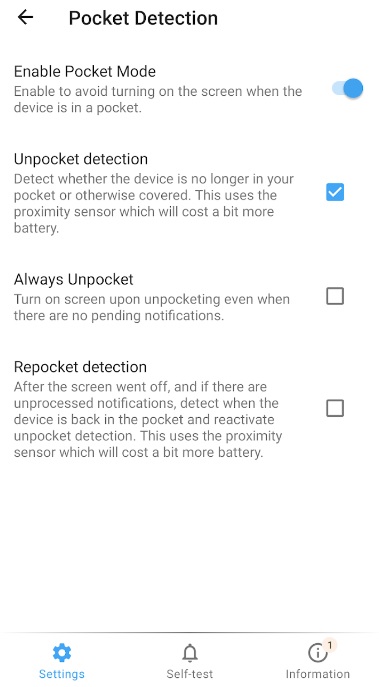**Detailed Caption:**

This image is a screenshot of a phone menu titled "Pocket Detection" prominently displayed in bold lettering at the top. A back button is located in the upper left corner. The menu contains several options related to pocket detection, each with its functionality and associated settings clearly listed.

1. **Enable Pocket Mode:** This option is turned on. It prevents the screen from turning on while the device is in your pocket.
   
2. **Unpocket Detection:** This option is enabled. It detects whether the device is no longer in your pocket or otherwise covered, utilizing the proximity sensor. This feature may consume slightly more battery.
   
3. **Always Unpocket:** This option is not checked. It would turn on the screen upon unpocketing, even when there are no pending notifications.
   
4. **Repocket Detection:** This option is not checked. It is designed to detect if the device is placed back in the pocket after the screen has turned off and there are unprocessed notifications. This feature also uses the proximity sensor, which can increase battery usage.

The text throughout the menu is presented in black or gray against a white background. At the bottom of the menu, there are three icons: a blue gear symbol representing the settings menu, a notification bell labeled "Self-test," and an information button depicted as a beige circle with the number one inside, indicating additional information is available.

Overall, this screenshot illustrates the various configurations available for pocket detection on a phone, providing users with several options to manage screen activity based on the device's proximity to the user’s pocket.